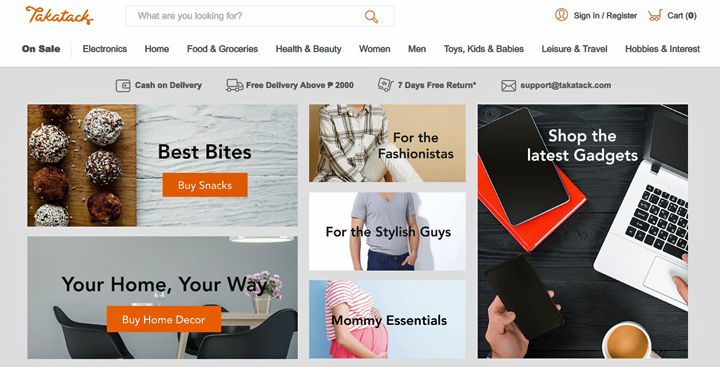The image showcases a user-friendly website interface featuring a header with a search bar and navigation links for various categories, including Electronics, Home, Food & Groceries, Health & Beauty, Women, Men, Toys, Kids & Babies, Leisure & Travel, and Hobbies & Interests. Below the header, there are colorful promotional banners encouraging users to take action, such as "Best Bites - Buy Snacks" with an orange button, "Buy Home Decor - Your Home, Your Way," "For the Fashionistas," "Shop the Latest Gadgets," and "Mommy Essentials for the Stylish Guys." The website emphasizes user convenience with services like cash on delivery, free delivery for orders above a specific currency amount, and a 7-day free return policy. The layout is straightforward and intuitive, making it easy for users to find what they need. Additionally, there is a support link to techostack.com for customer assistance.